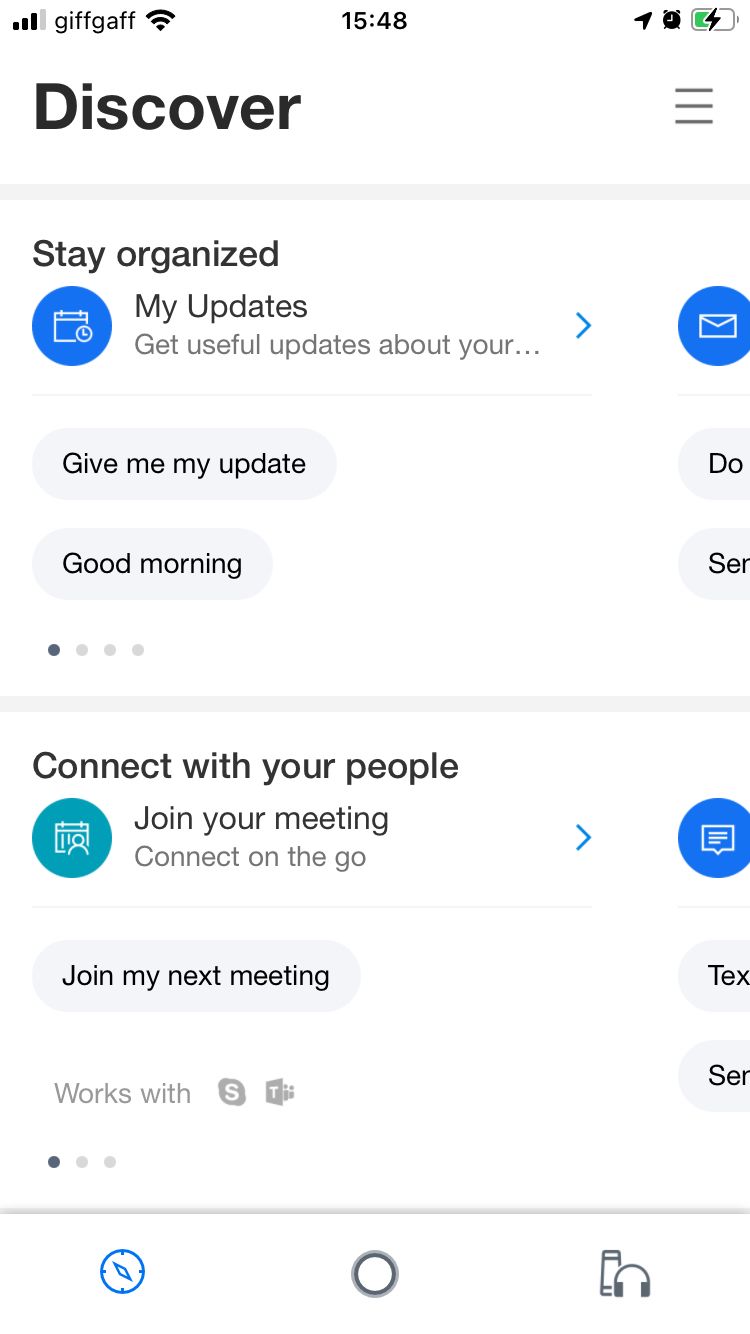Screenshot Description:

The image is a narrow, elongated screenshot likely taken from a smartphone. At the very top, there are several status icons, including a phone signal displaying three out of four bars, the text "GIFFGAFF" indicating the service provider, a Wi-Fi signal icon, and the time displayed in military format as "15:48". Following these are additional symbols: a right arrow, a cat-shaped box (possibly an alarm clock with a black face) which is very small, and a half-full battery icon.

Beneath this status bar, there is a bold black "Discover" heading with a three-line menu bar icon next to it. A thin gray line separates this header from the content below. The first section titled "Stay Organized" features the subheading "My Updates" and prompts the user with "Get Useful Updates About Your" followed by a right arrow and an email symbol. The next line reads, "Give Me My Updates Due" and "Good Morning S-E-R" followed by four dots.

The next section is titled "Connect with Your People" and offers several options: "Join Meeting" and "Connect on the Go" indicated with a right arrow and a circle with a text box icon. There is an option labeled "Join My Meeting" followed by the text "T-E-X" and a combination of a dollar sign and another icon labeled "S-E-R".

At the bottom, there are three dots, a gray line possibly indicating a separator, a settings symbol, a circle, and an earphone image.